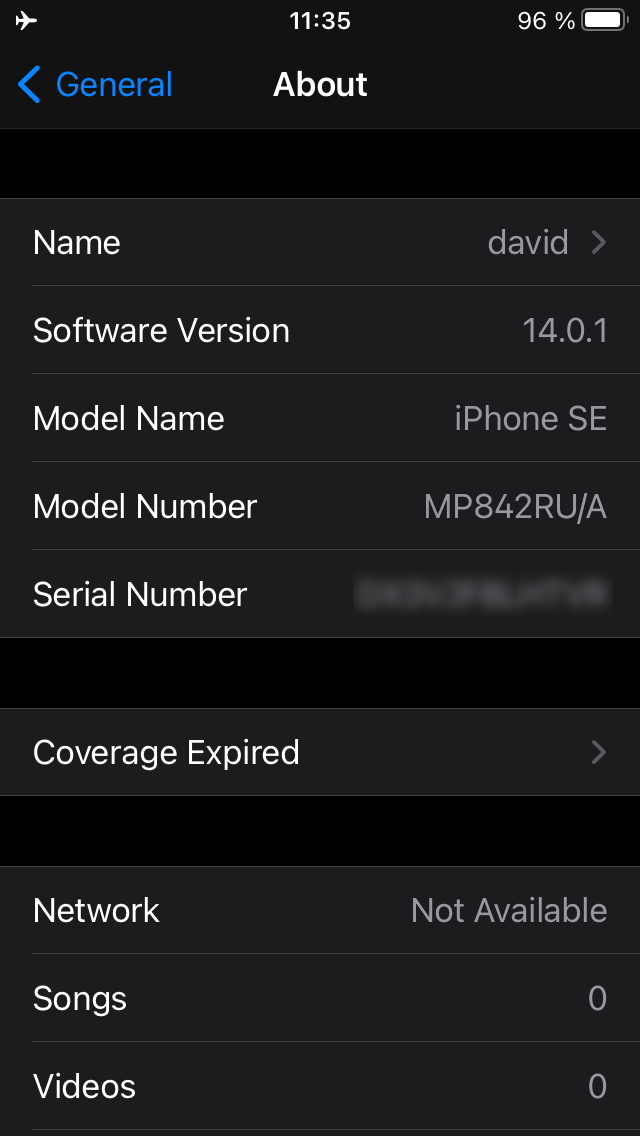The image depicts a smartphone screen displaying the "About" section under the "General" settings, with the device in flight mode. It is currently 11:35 AM, and the battery life is at 96%. The top navigation bar shows "General" in blue on the top-left corner with a back arrow, and "About" in white centered at the top.

The screen features a vertical list of device information on a black background, with text primarily in white. The details are as follows:
- Name: "David" (displayed in gray next to the label "Name")
- Software Version: "14.0.1" (in gray)
- Model Name: "iPhone SE" (in white)
- Model Number: "MP842RU/A" (in gray)
- Serial Number: (information grayed out)
- Coverage Status: "Coverage Expired"
- Network: "Not Available" (in gray)
- Songs: "0"
- Videos: "0"